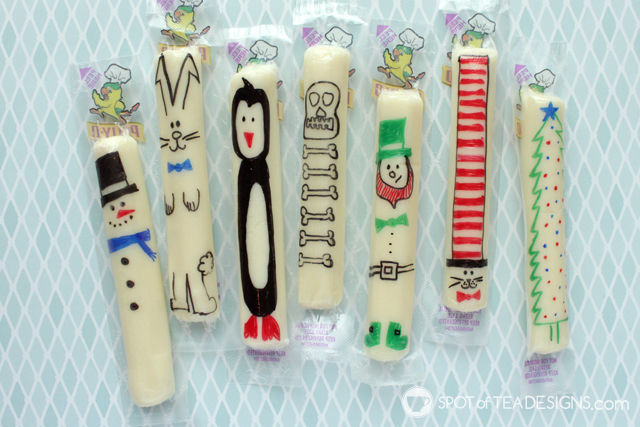This up-close photo features seven individually wrapped string cheese packages, arranged on a blue diamond-patterned tablecloth. Each cheese stick package has been turned to display unique children's drawings, transforming the back of each pack into a canvas. Starting from the left, the first cheese stick showcases a snowman with a black hat, blue scarf, and three buttons. Next is an Easter Bunny wearing a blue bow tie. The third depicts a penguin, detailed with black and white coloring, an orange beak, and matching feet. Following is a skeleton with a skull and six bones drawn beneath it. The fifth cheese stick highlights a leprechaun with a red beard, green hat, bow tie, and shoes, including a belt. To its right, there is a cat with a very tall, red-striped top hat resembling the Cat in the Hat, its face drawn near the bottom of the package. The final cheese stick portrays a Christmas tree, filling the entire height of the packaging. Additionally, there is a small label in the bottom right corner of the image, featuring a coffee cup and the text "spotoftdesigns.com" in a white circle. Purple lettering that reads "peel here" is visible near the top left corner of each string cheese package.